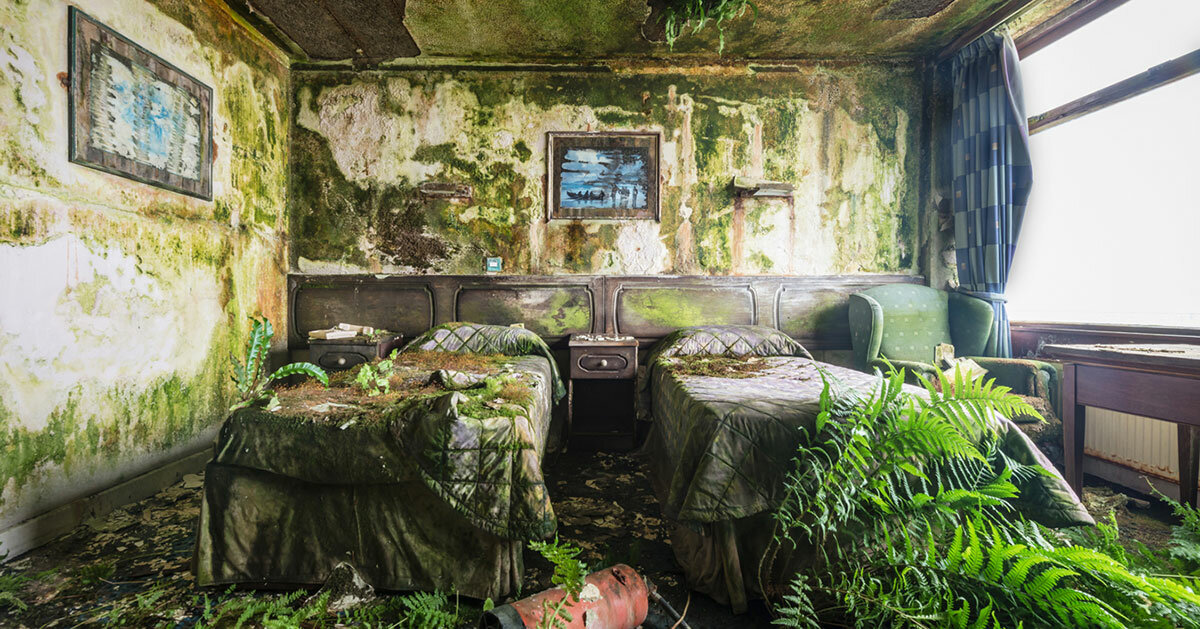This color photograph depicts a dramatically decayed and abandoned bedroom, potentially once part of a hotel. The room is overtaken by nature, with green stains and brown smears marking the cracked, mildewed walls. Ferns and other plants grow up from the floorboards, with vines draping from the ceiling. Dominating the right wall, a large rectangular window allows light to wash over the room, its blue curtain—the cleanest object in sight—pulled partially to one side.

Against the back wall, a long, built-in wooden headboard runs beneath the window. It spans the width of the room and serves two small beds, separated by a small nightstand with a drawer. The bedspreads are moldering and covered in debris; the left bed hosts a plant, while a large fern grows at the foot of the right bed. A blue, wing-back armchair sits stained and dirty next to the right bed.

On the left wall, an old, dirty framed print hangs, barely discernible through the layers of mildew and grime. Another small picture rests between the bed heads, though its details are obscured by decay. Near the headboard, a tipped-over fire extinguisher lies surrounded by ferns adding to the sense of desolation and abandonment. The atmosphere recalls scenes from disaster-stricken areas or forgotten ruins, underscored by the haunting absence of an outside landscape visible through the translucent window.